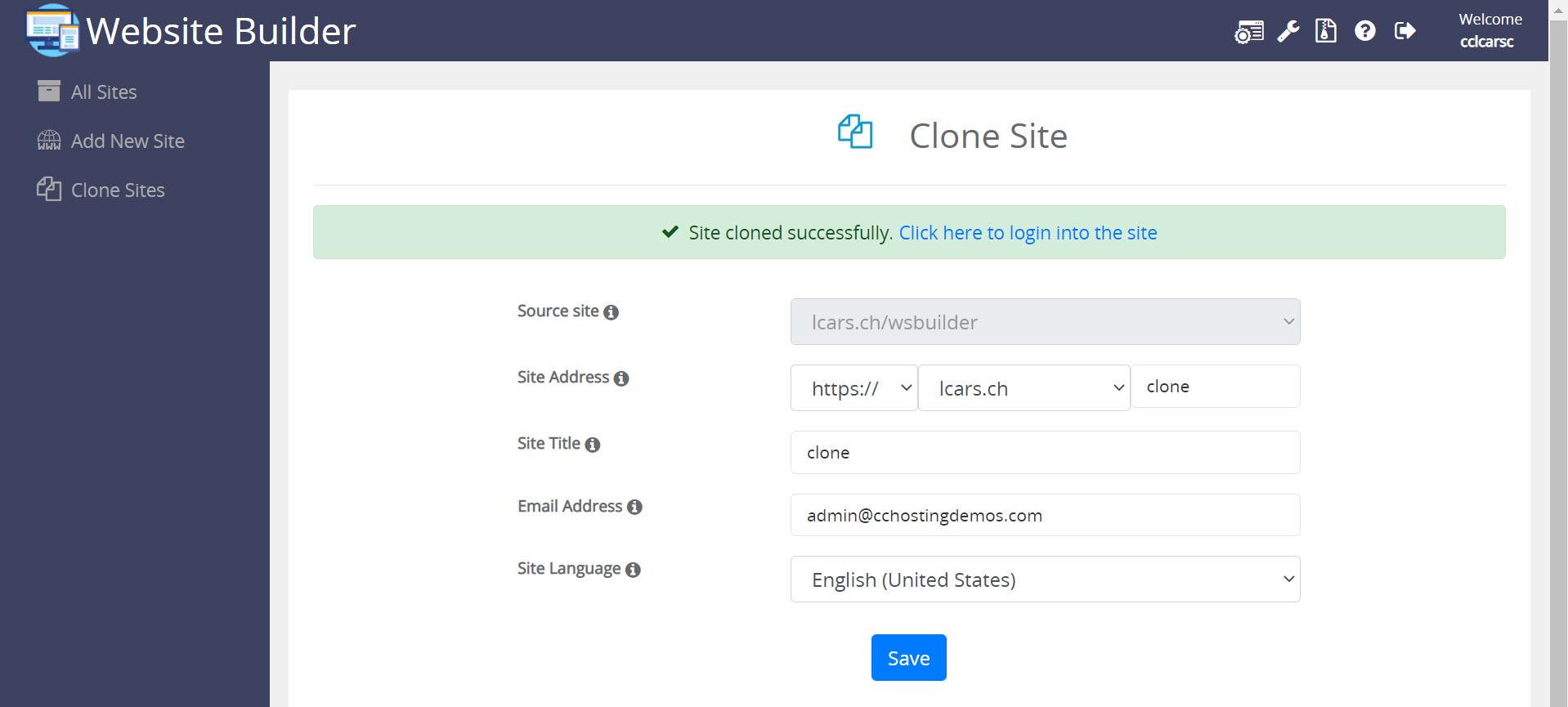This is a detailed screenshot of a website builder interface. The primary background color is dark navy blue, featured on the header bar and the left navigation menu. The main content area within the website design section has a light gray background, with the actual workspace showcased in white. A vertical scroll bar is present on the far right.

In the top left corner of the header bar, there is a light blue circle containing drawings of a computer monitor and a mobile device screen, representing the website builder's logo. To the right of the logo, the text "Website Builder" is displayed in white. Further along this top bar are five icons, followed by a "Welcome" message and the user's username.

On the left-hand side, the navigation bar presents options like "All Sites," "Add New Site," and "Clone Site," all set against the dark navy background. The current screen focuses on the "Clone Site" feature, displayed in the main white content area. Central to this area is a title "Clone Site," illustrated with two pages having their top left corners folded in blue.

Immediately below the title, there is a horizontally-aligned mint green bar with a success message "Site cloned successfully." A clickable blue link within this bar reads "Click here to log into the site."

Underneath the success message are five rows of settings. The first column labels these settings as "Source Site." Each row includes various input elements—text boxes, drop-down menus, and checkboxes. Here’s a breakdown of these rows:

1. Drop-down text bar for selecting the source site address.
2. A dropdown for choosing the protocol (http or https).
3. A dropdown for selecting the site name, such as "icars.ch."
4. Text boxes where the cloned site title, email address (admin@cchostingdemos.com), and site language (English - United States) can be specified.

Beneath all these settings, there is a blue button with "Save" written in white text, enabling the user to save the cloned site settings.